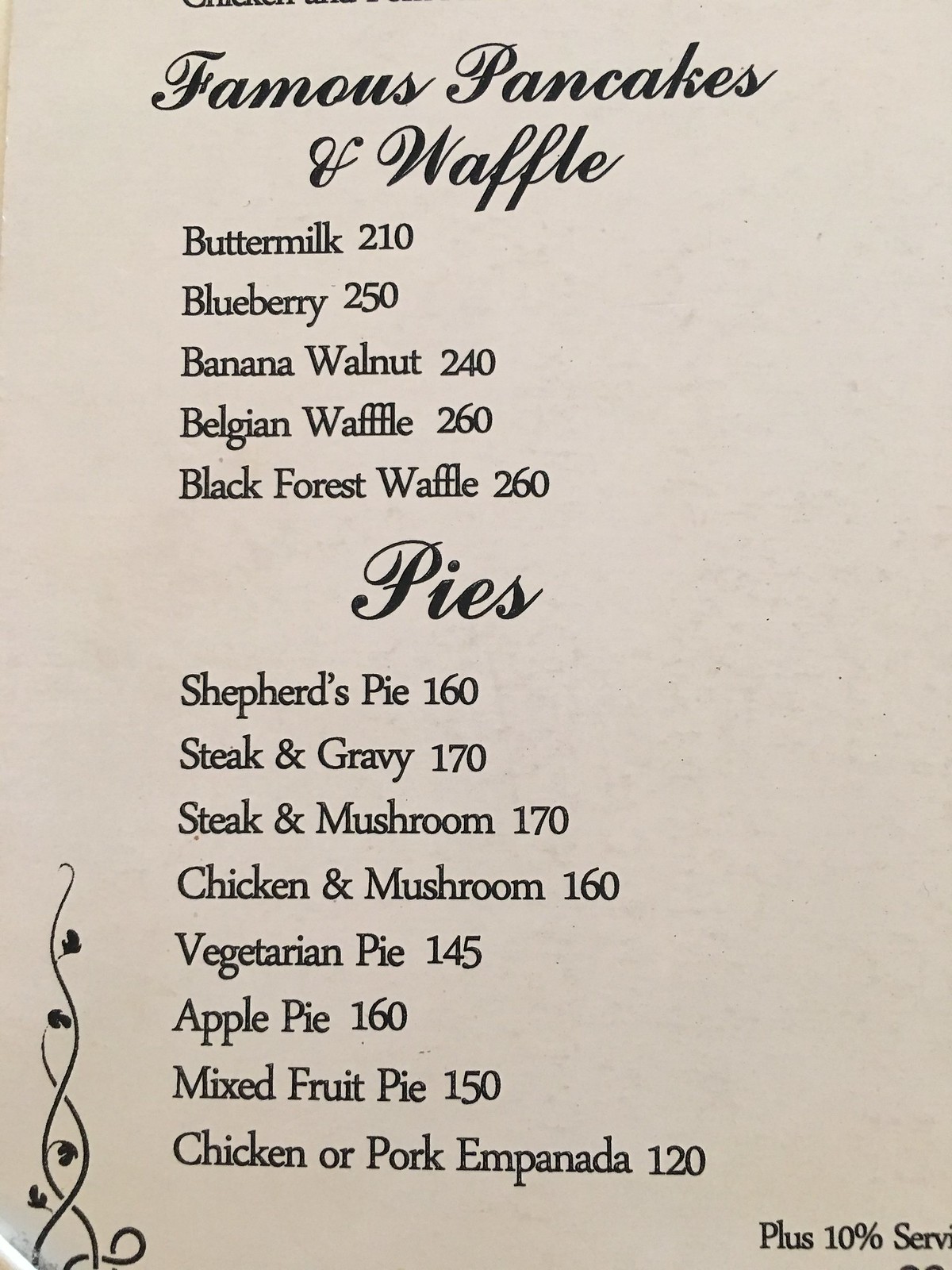The image showcases a menu titled "Famous Pancakes and Waffles." The top section lists various pancake and waffle options including Buttermilk, Blueberry, Banana Walnut, Belgian Waffle, and Black Forest Waffle, with prices ranging from $2.10 to $2.60. Midway down, the menu transitions to the "Pies" section, offering a variety of savory and sweet choices such as Shepherd's Pie, Steak and Gravy, Steak and Mushroom, Chicken and Mushroom, Vegetarian Pie, Apple Pie, Mixed Fruit Pie, and Chicken or Pork Empanada, priced between $1.20 and $1.70. The menu is printed on plain paper with all text in black type.